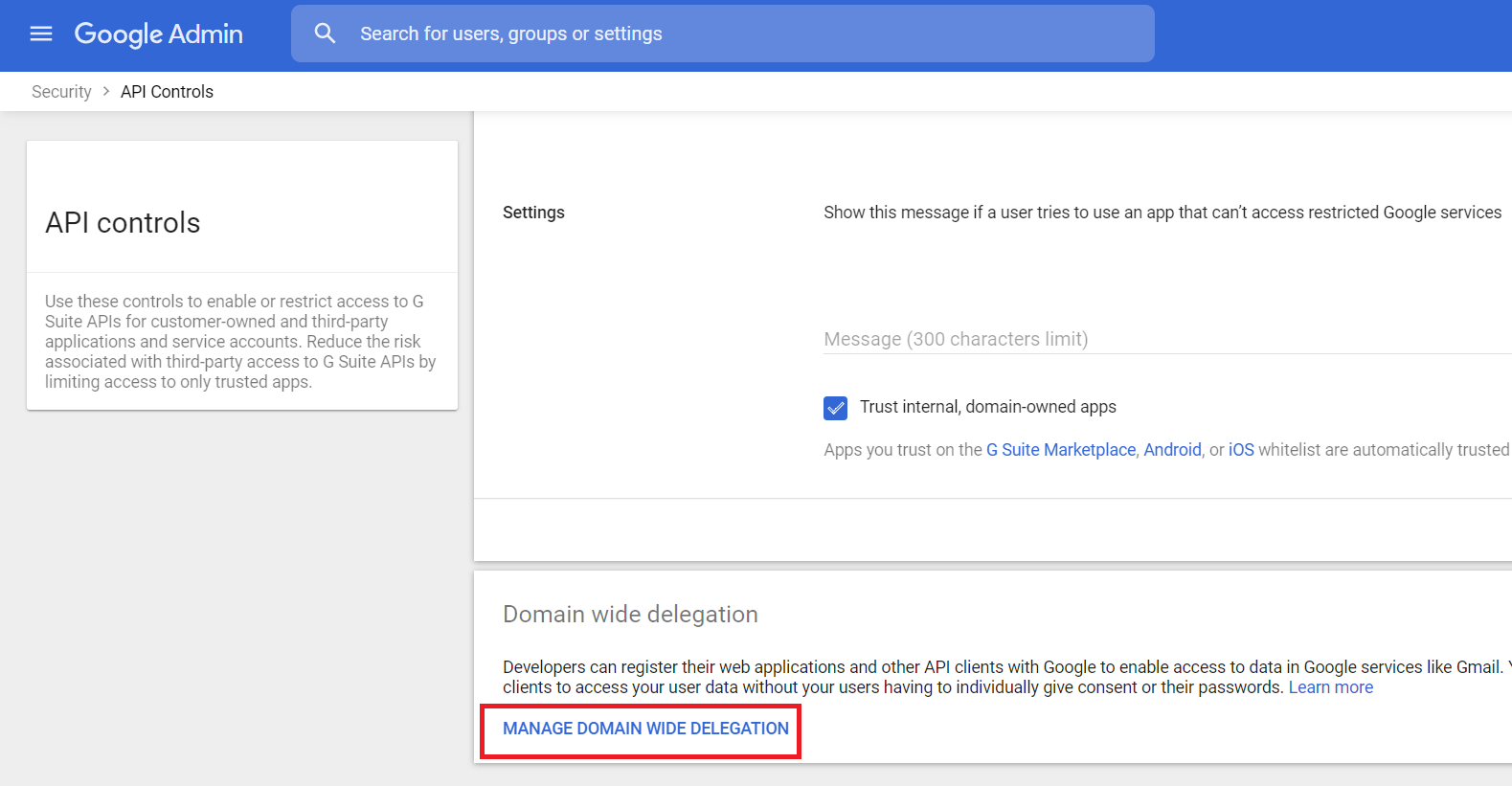The webpage features a blue header that contains a three-bar hamburger menu icon located on the left side. To its right, in white text, is the label "Google Admin." Overlaying the header is a semi-transparent rectangular bar with white text and a magnifying glass icon that reads "Search for Users, Groups, or Settings."

The main content area has a white background. Below the header, on the top left of the page, the word "Security" appears in a gray font, followed by an emphasized "API Controls" with a caret pointing toward it. Below this section, a vertical gray column provides additional context about API controls, including a paragraph describing their function.

The main portion of the page is headed by the word "Settings," which includes various options. One setting titled "Show this message if a user tries to use an app that can't access restricted Google services" is followed by a "Message 300 Characters Limit" label and a check box. At the bottom of the page, under the section "Domain-Wide Delegation," there's a button labeled "Manage Domain-Wide Delegation" in a blue hyperlink style, highlighted with a red rectangle.